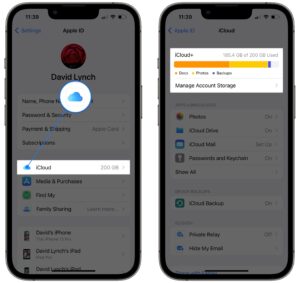In this screenshot of an Apple iPhone, the Settings app is open to display the user's Apple ID information. The name "David Lynch" is prominently visible at the top of the screen. Various categories are listed under the Apple ID settings, including "Name, Phone Numbers, Email," "Password & Security," "Payment & Shipping," "Subscriptions," "iCloud," "Media & Purchases," "Find My," and "Family Sharing." 

David has selected the "iCloud" option, revealing a detailed view of their iCloud storage usage. It indicates that David subscribes to a 200 GB iCloud+ plan, which is approximately 90% full. While a significant portion of the storage is used for photos, there are additional large files contributing to the storage consumption. 

The iCloud section also shows that David’s photos, iCloud Drive documents, and iCloud Mail are backed up to iCloud. Additionally, it’s noted that David has multiple Apple devices connected to his iCloud account, including this iPhone, an iPad, and another unspecified device.